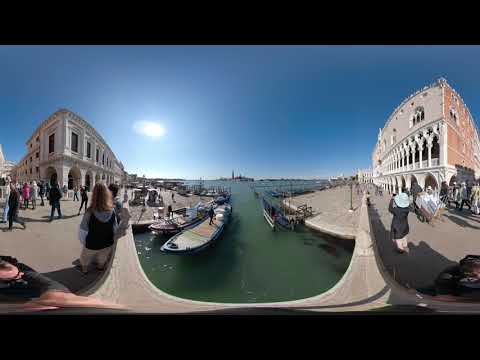This photograph captures a picturesque scene in Venice, Italy, showcasing its iconic architectural charm and vibrant atmosphere. Dominating the left side of the image is a majestic historic building, distinguished by its numerous columns and a small window perched high above. The central focus of the image is a serene green canal, with a classic gondola gracefully gliding towards a curving embankment. The U-shaped sidewalk around the canal, bustling with tourists, offers panoramic views of both the water and a distant cityscape. The sky overhead is a brilliant blue, adorned with a solitary cloud and bathed in bright sunlight, enhancing the beauty of the old tan-colored buildings that frame the scene. These buildings, marked by their arched openings, add to the Venetian ambiance, where the elegant gondolas and lively crowds further enrich the lively, timeless charm of this stunning locale.